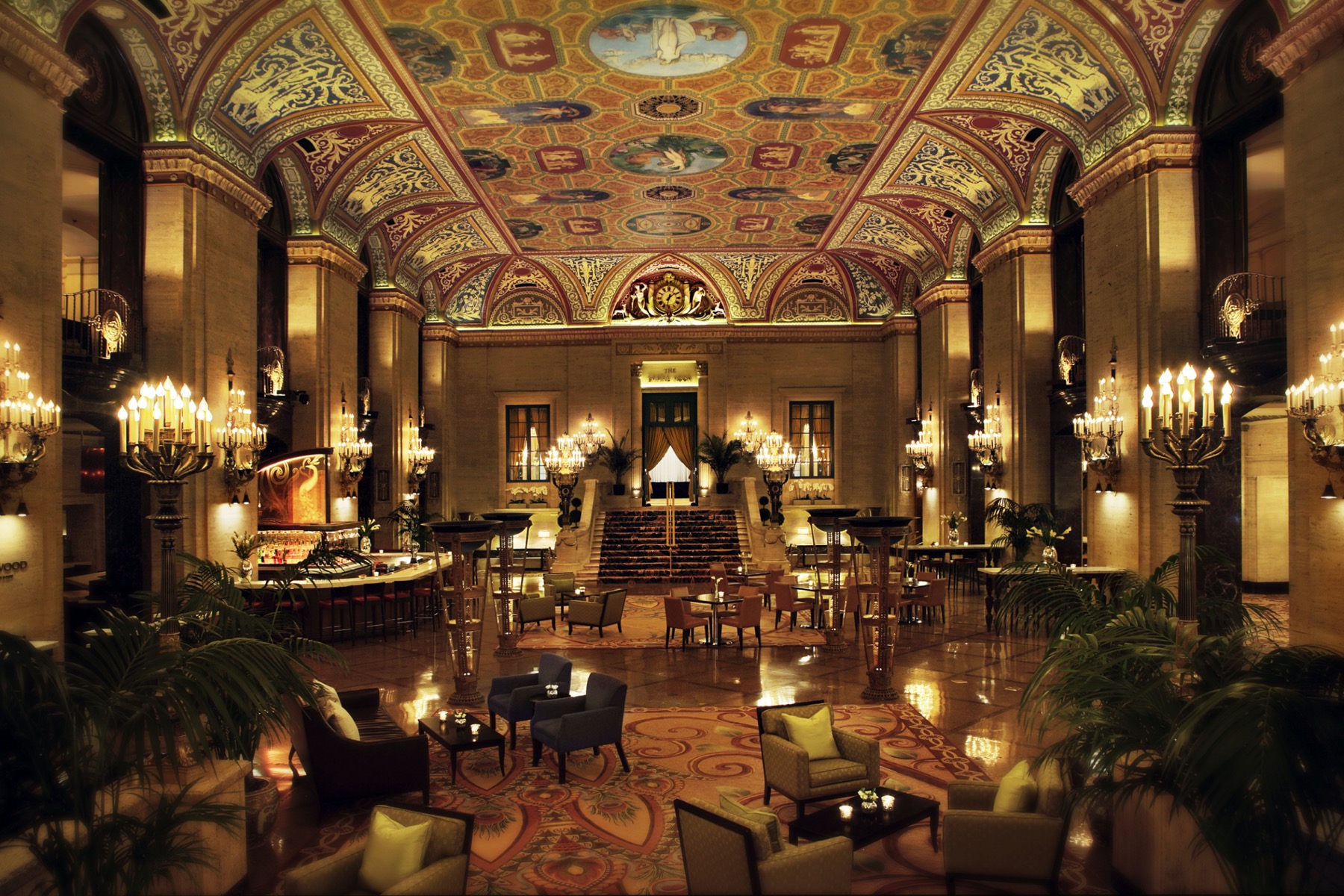This image showcases an elaborate, opulent lounge area, possibly from an iconic hotel in Chicago, designed in a Victorian style. The spacious room is adorned with a mix of tan, brown, and blue chairs, all surrounding glass and brown tables. A large tan and red area rug adds warmth to the floor. The ceiling is intricately designed with golden hues and vibrant paintings of reds and blues, complemented by strikingly tall archways and richly detailed tile work. Crystal chandeliers, pedestal lights, and black bowl lamps on conical frames provide a warm and inviting ambiance. Lush plants add a touch of greenery throughout the room. The left side features a small bar and a reception desk, while the far end houses a staircase leading up to a doorway. The walls, constructed from brick, are adorned with candle stands that further illuminate the space. The overall atmosphere exudes luxury and sophistication, making it an impressive and memorable space.